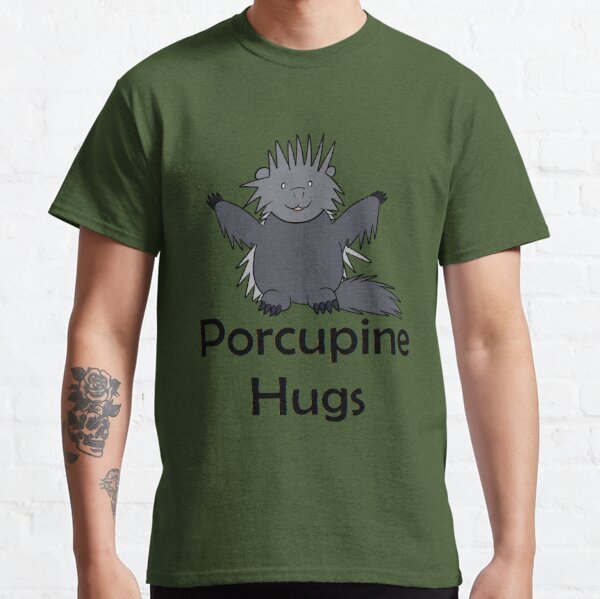This photograph features a white male model wearing a round neck, short sleeve, dark khaki green t-shirt that is cut off just at his Adam's apple and at his hips. The focal point of the shirt is a cute, stylized cartoon porcupine depicted in dark grey, black, and light grey with white eyes, spiky hair, a fluffy tail, and cute claws. The porcupine has its arms spread out as if offering a hug. Below the character, in black text, it reads "Porcupine Hugs." The model’s right arm is adorned with visible black ink tattoos, including a skull on his forearm and another tattoo on his wrist. The image is set against a white background, emphasizing the t-shirt and giving it a professional, online shopping vibe, reminiscent of what one might find on Etsy or similar websites.